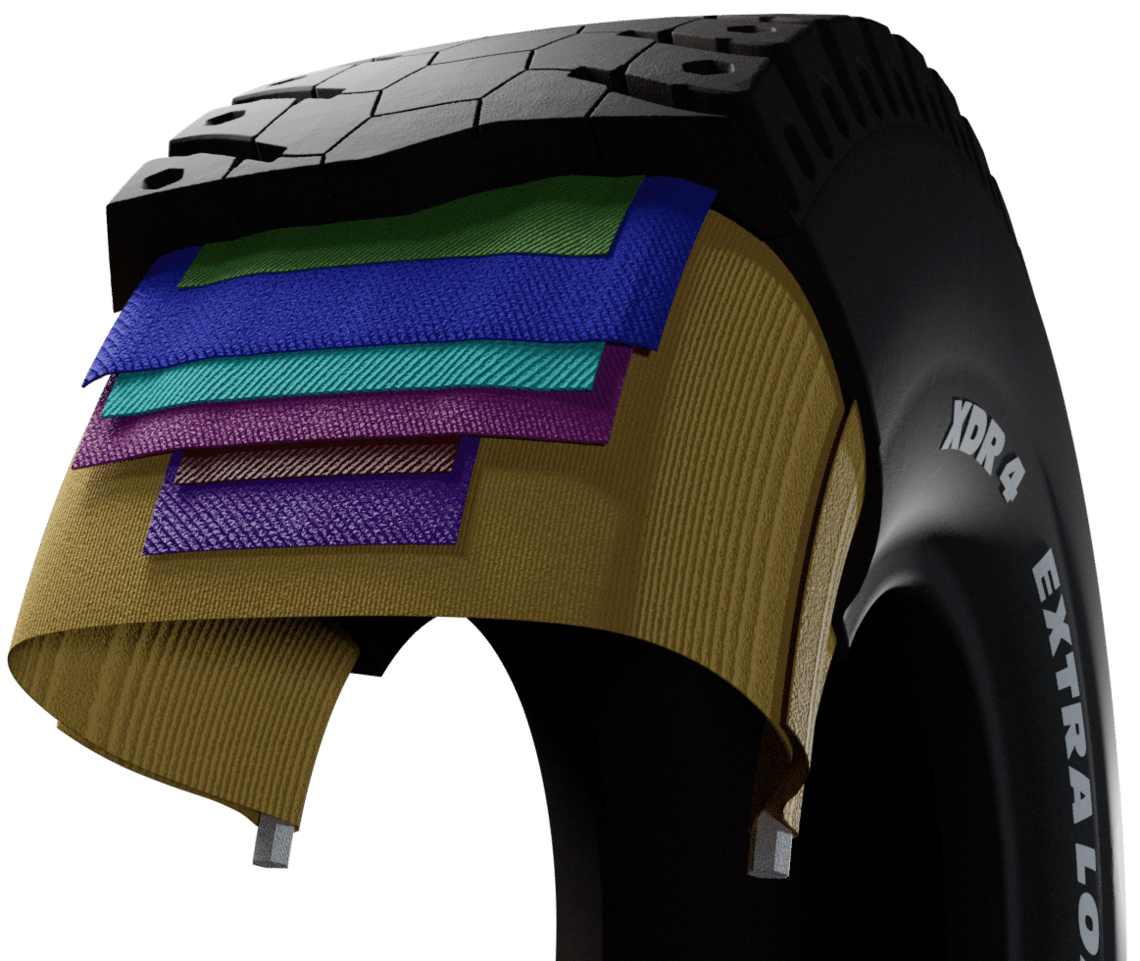This image is a computer-generated, artist's depiction of a cutaway radial tire for a pickup truck. The tire, made of thick black rubber, has been sliced open to reveal its intricate internal structure. Displayed along the sidewall, partially visible text reads "XDR 4 extra LO," before being cut off. The inner composition showcases multiple distinct layers, each color-coded to demonstrate the materials used. Starting from the outermost layer, there's a thin brown-gold layer, followed by a purple layer, a narrower brown layer, a wider fuchsia layer, and successive layers of teal, blue, and a smaller green layer. These layers appear woven together in various patterns to indicate different types of materials, possibly steel and fabrics, contributing to the tire's sturdiness and puncture resistance. The depiction provides a detailed understanding of the complex construction involved in making a steel radial tire for heavy-duty vehicles.